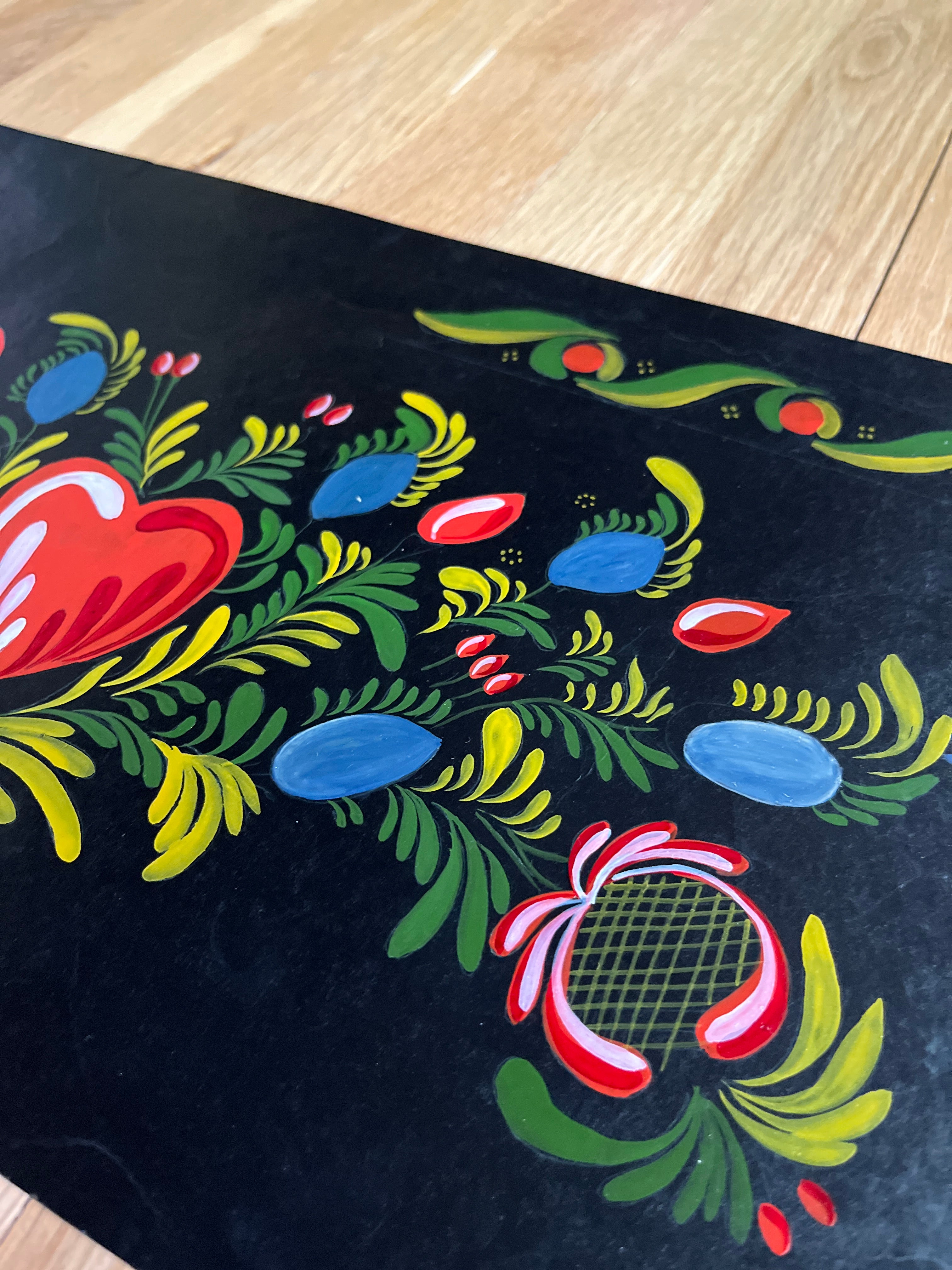The image depicts a wooden table or floor surface featuring a black mat adorned with a vibrant, floral design. The pattern includes heart shapes intertwined with green and yellow leaves, as well as swirling designs. Sprinkled across the mat are clusters of four yellow dots and blue shapes resembling plums or fruits, adding to the colorful, intricate floral motif. The mat's background remains black to highlight the diverse palette of greens, blues, yellows, and accents of dark red and pink. The black mat spans across the angular wooden surface, which is wider on the right and narrower on the left.